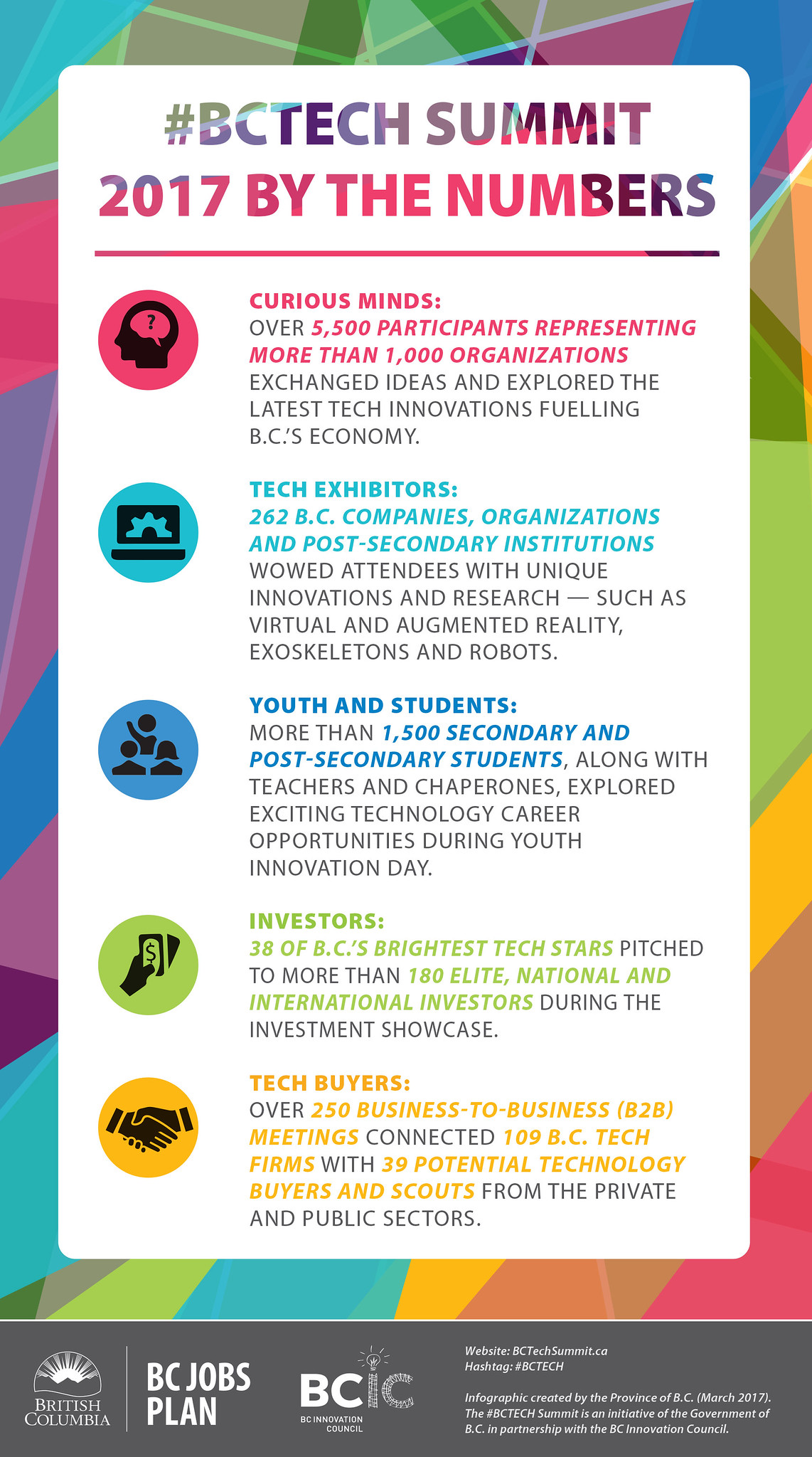This vibrant promotional poster from the BC Tech Summit 2017 showcases key statistics and achievements with a multicolored backdrop featuring hues of blue, purple, green, yellow, red, and other colors flowing together. The prominent white rectangle in the middle contains all the text, starting with a hashtag followed by "BC Tech Summit 2017 by the Numbers," written in a darker color. 

Under this heading, there are five sections highlighted with bold colors and corresponding icons on the left-hand side, each section boasting specific achievements:

1. **Curious Minds** (Red): Depicted with a mind icon, this section details that over 5,500 participants from more than 1,000 organizations exchanged ideas and explored the latest tech innovations fueling BC's economy.

2. **Tech Exhibitors** (Light Blue): Represented by a computer icon, it mentions that 262 BC companies, organizations, and post-secondary institutions impressed attendees with unique inventions and research, including advancements in virtual and augmented reality, exoskeletons, and robotics.

3. **Youth and Students** (Darker Blue): Illustrated with a student icon, this category highlights how more than 1,500 secondary and post-secondary students, along with teachers and chaperones, discovered exciting technology career opportunities during Youth Innovation Day.

4. **Investors** (Green): Marked with a dollar sign icon, this segment notes that 38 of BC's brightest tech stars pitched their ideas to over 180 elite national and international investors during the investment showcase.

5. **Tech Buyers** (Yellow): Accompanied by a handshake icon, it states that over 250 business-to-business meetings facilitated connections between 109 BC tech firms and 39 potential technology buyers and scouts from both the private and public sectors.

At the bottom, in yellow, it prominently displays the "BC Jobs Plan". To the left of the categories, there's the BC insignia against a black backdrop with "British Columbia, BCIC" written underneath.

Overall, the poster highlights the robust participation and dynamic innovations presented at the summit, illustrating its significant impact on the BC tech industry through a rich, colorful visual presentation.